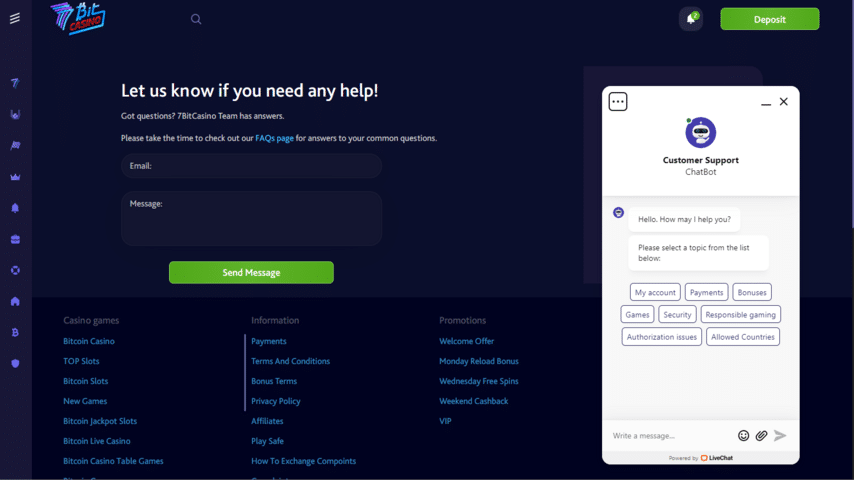**Detailed Caption:**

The image displays a page from BitCasino. At the top left corner, the program's name, BitCasino, is prominently featured. Beside it is a helpful prompt: "Let us know if you need any help. Got questions? 7BitCasinoTeam has answers. Please take the time to check out our Frequently Asked Questions page for answers to your questions."

The central section of the page includes an email field, a message field, and a "Send Message" button, facilitating easy communication with the support team. An intuitive magnifying search button is located at the top edge of the image for quick navigation.

On the left side of the interface, a row of icons provides access to various functions and sections. At the bottom of the page, there is a list of linked text pertaining to different categories and game types, including Casino Games, Bitcoin Casino, Chop Slots, Bitcoin Slots, New Games, Bitcoin Jackpot Slots, Bitcoin Live Casino, Bitcoin Live, and several other games.

To conclude, there is a note of appreciation: "Thank you for watching. Please subscribe to our channel." This message is reiterated, emphasizing the call to action for audience engagement.